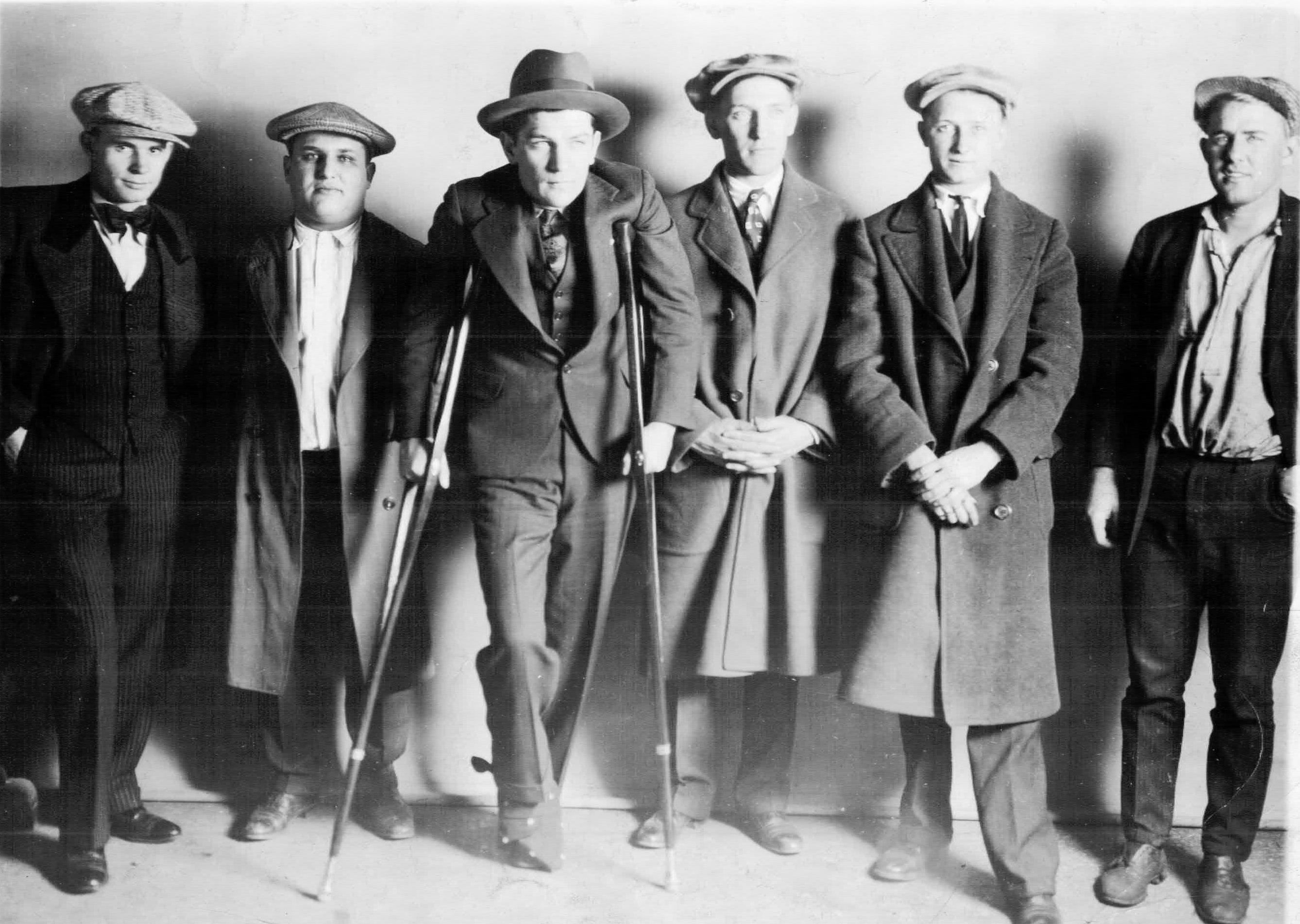This black-and-white photograph, likely taken in the early 20th century, depicts six men standing in a line against a textured wall. Their attire consists mostly of suits accented with various styles of hats popular during the era. Most of the men wear jackets or peacoats, complementing their vests and ties, with one man sporting a bow tie and another noticeably without any neckwear. The third man from the left stands out as he leans on crutches, suggesting an injury to his right leg, and wears a white-brimmed hat that contrasts with the newsboy and fabric caps worn by the others. The last man appears more casually dressed with a loose-fitting shirt and a short open jacket. The photograph, characterized by its grainy texture and slightly out-of-focus appearance, exudes a historical ambiance, capturing a stoic, unsmiling moment in time.